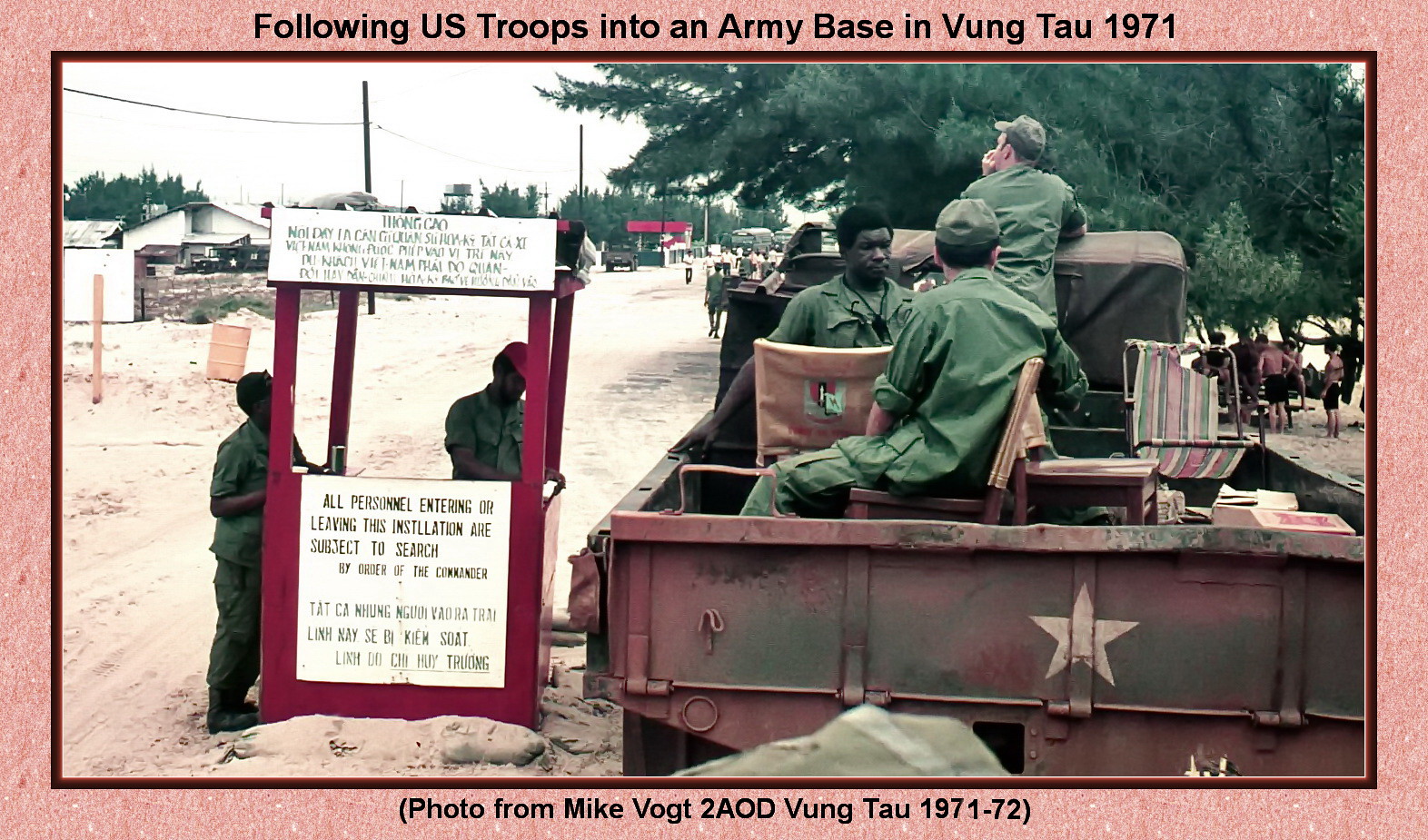This detailed photograph, likely from a publication or website, depicts U.S. troops and military activity at an army base in Vung Tau, Vietnam, dated 1971-72. In the foreground, several soldiers dressed in green army fatigues are either seated or standing in the back of a military jeep marked with a white star. Adjacent to the jeep stands a distinctive red wooden booth with a sign that reads, "All personnel entering or leaving this installation are subject to search by order of the commander." Inside and around this booth, additional soldiers can be seen. The scene captures a sandy area with scattered trees and a road, notable in the background is a large bus and some buildings. Additionally, there are civilian men in casual clothing, possibly in swim trunks, walking down the street or congregating under a tree, enhancing the contrasting elements of military order and casual civilian life. The photograph is framed with a peach-colored border, and inscribed at the top is "Following U.S. troops into an army base in Vung Tau, 1971," and "Photo from Mike Vogt, 2AOD, Vung Tau, 1971-72" at the bottom.